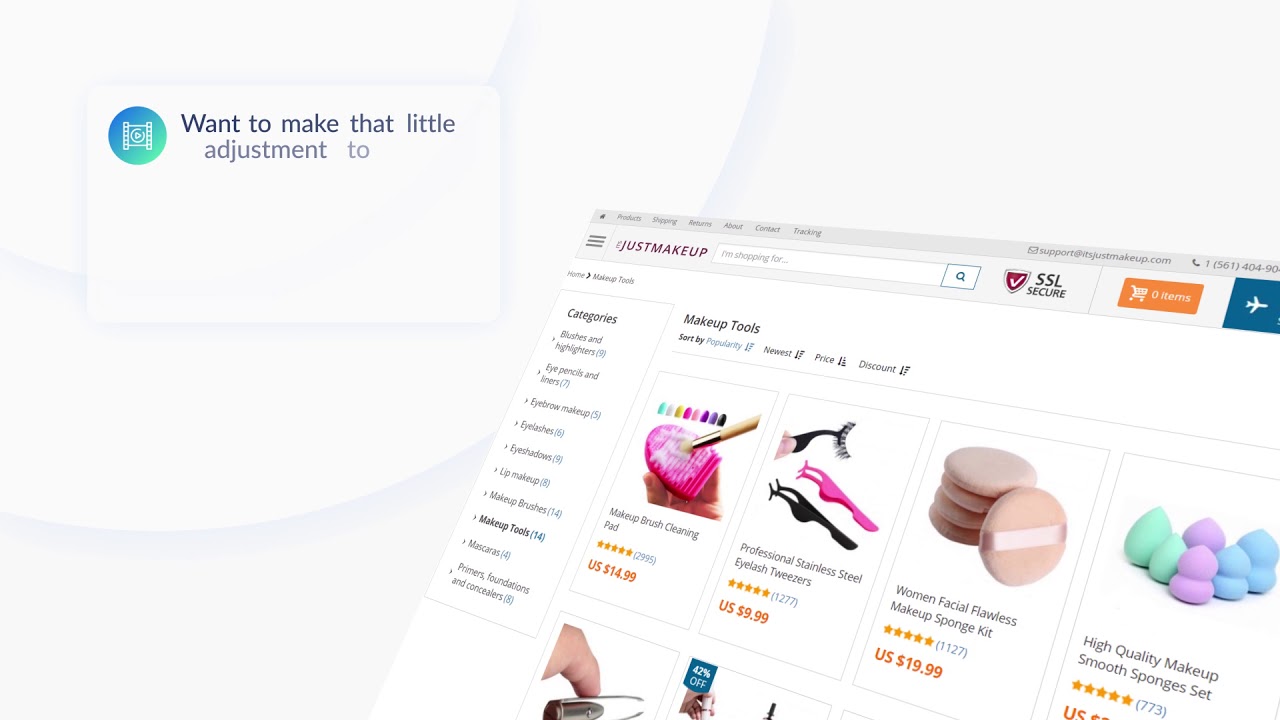A detailed screenshot displays an online ordering interface focused on cosmetics. The header reads "Want to make that little adjustment?" in white font against a subtle gradient background. To the side, categories are listed under "Just Makeup," which include "Makeup Tools." The view is angled, showing a side perspective of various makeup products such as sponges, eyelash applicators, and tweezers. Each item appears in organized sections with detailed descriptions and prices. The interface also indicates a secure checkout process, ensuring the safety of the purchase.